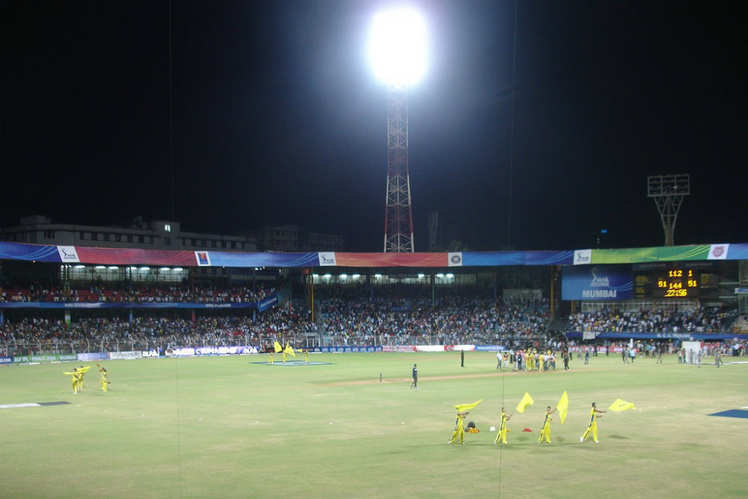The image depicts a vibrant nighttime sporting event in a large outdoor stadium. Bright lights mounted on towering scaffolding illuminate the entire scene. The packed stadium has two tiers of seating, adorned with colorful banners displaying various sponsor logos, though they are somewhat indiscernible from a distance. Along the top rim of the stands, a patterned banner featuring blue, white, and red stripes provides a decorative touch.

Prominently displayed is a black electronic scoreboard with bright yellow numerals reading 112, 181, and 51, next to a blue banner that reads "Mumbai" accompanied by what might be the country flag symbol. Situated in the background left is a large, somewhat obscured industrial or institutional building.

On the meticulously short-cut green field, groups of people are spread out. Many of them, wearing yellow jumpsuits, appear to be participating in a coordinated performance, enthusiastically waving yellow flags. Others, dressed in different attire, are scattered around, with a concentration of people in the middle and towards the right side of the field. The stadium is filled with spectators, their faces indistinct, contributing to the lively and celebratory atmosphere of the event.